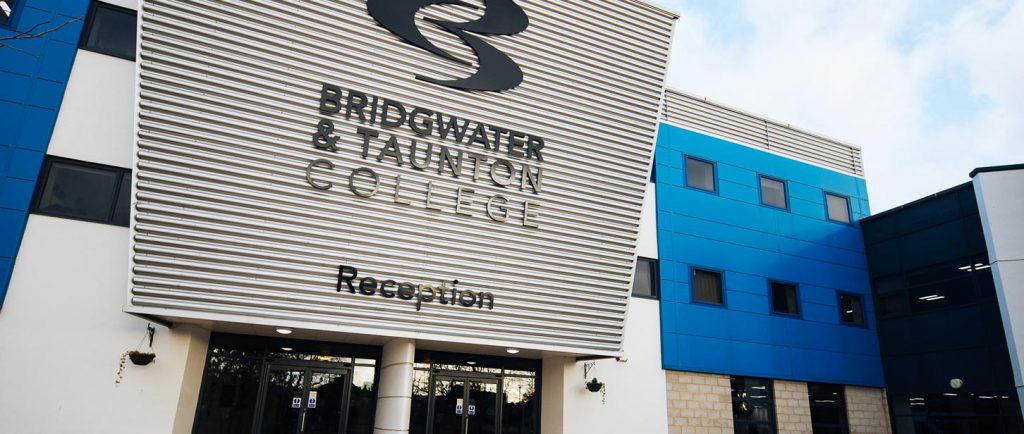The image showcases the reception entrance of Bridgewater and Tarkton College, characterized by its modern 70s-inspired architecture. Central to the entrance is a circular pylon flanked by glass doors on either side. The facade features a distinctive chimpanzee-shaped wall with a ribbed pattern, prominently displaying the college's logo—a stylized combination of a '3' and a 'C' in black. Beneath the logo, the name "Bridgewater and Tarkton College" is inscribed, with "Reception" written below it.

On either side of the main entrance, the building is framed by white walls adorned with black square windows. To the right, a bright blue section of the facade houses six additional square windows, adding a splash of color to the scene. The left side mirrors this blue element, contributing to an asymmetrical yet cohesive design. Hanging plants by the doors add a touch of greenery, and the glass surfaces reflect the cloudy, foggy sky above, enhancing the photograph's atmospheric quality. The building's textured detailing, such as the horizontal lines on the silver signage, further accentuates its modern aesthetic.